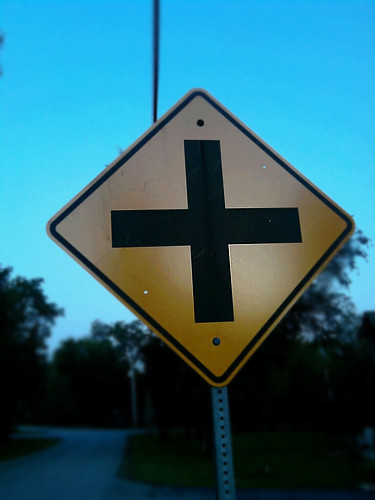This image captures a diamond-shaped, gold-colored traffic sign positioned on a metal stand along a roadway. The sign features a prominent, thick black cross in the center, encased by a black outline, likely signaling an approaching intersection. The scene is dimly lit, giving it a somewhat dark and moody atmosphere. Above the sign, power lines stretch across the sky, adding to the industrial aesthetic. Large trees border the road, but no buildings or houses are visible due to the insufficient light. The road ahead is partially visible, with smaller roads branching off into the darkness, further emphasizing the sign's warning of an upcoming intersection.